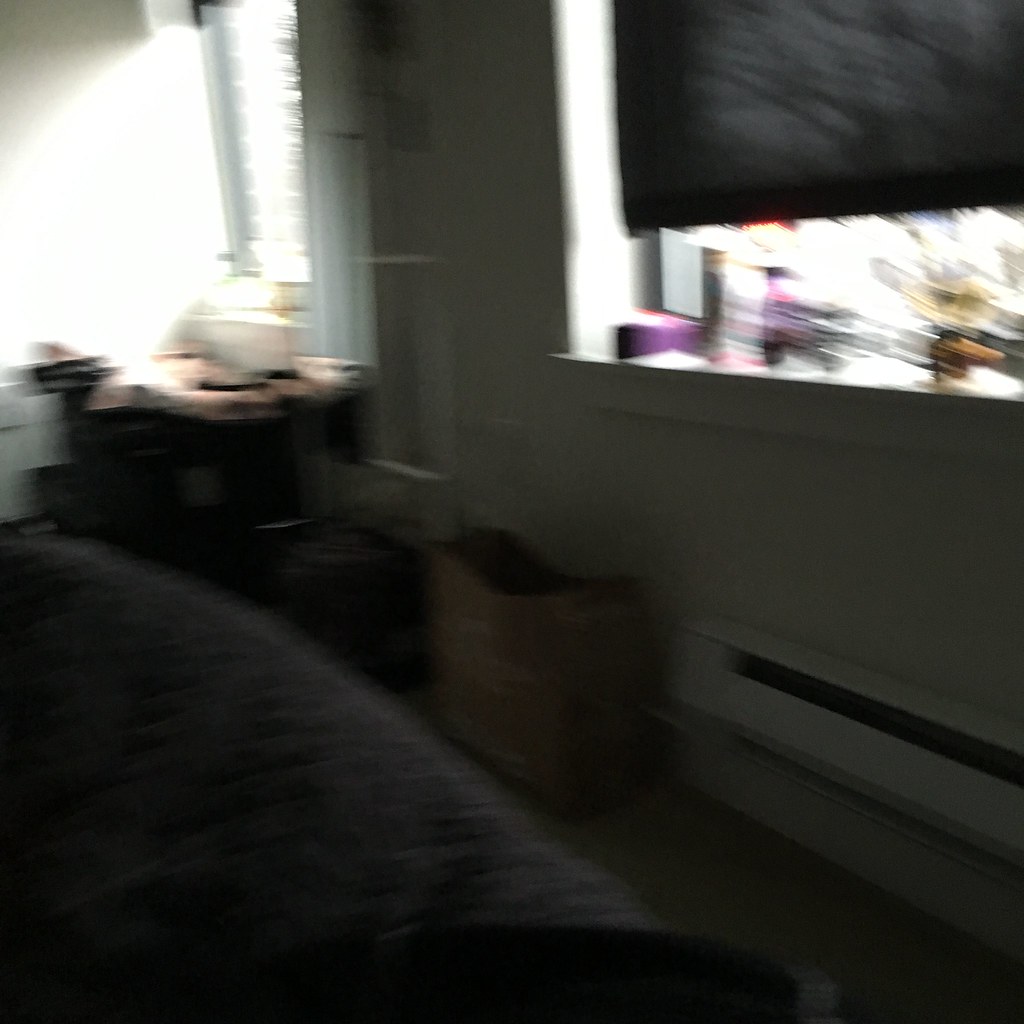This photograph, although blurry, captures the corner of someone's bedroom. Central to the image is a slightly raised, canvas roller shade, allowing light to stream in from a window. The window sill beneath the shade is cluttered with various items. Below the sill, a white radiator or heating element is mounted on the wall, with a large brown open container on the floor, possibly a basket or a grocery bag. The wall is white, and the floor is covered with a beige carpet. To the right, partially visible, is a grey bedspread, suggesting the photo was taken from the bed. Off in the corner, there is a table or desk without a chair, hinting it might be more decorative than functional. Another window is situated to the left, contributing additional light. A black object, likely the edge of the bed, is visible in the bottom left corner. Overall, the room appears somewhat disorganized and lived-in.